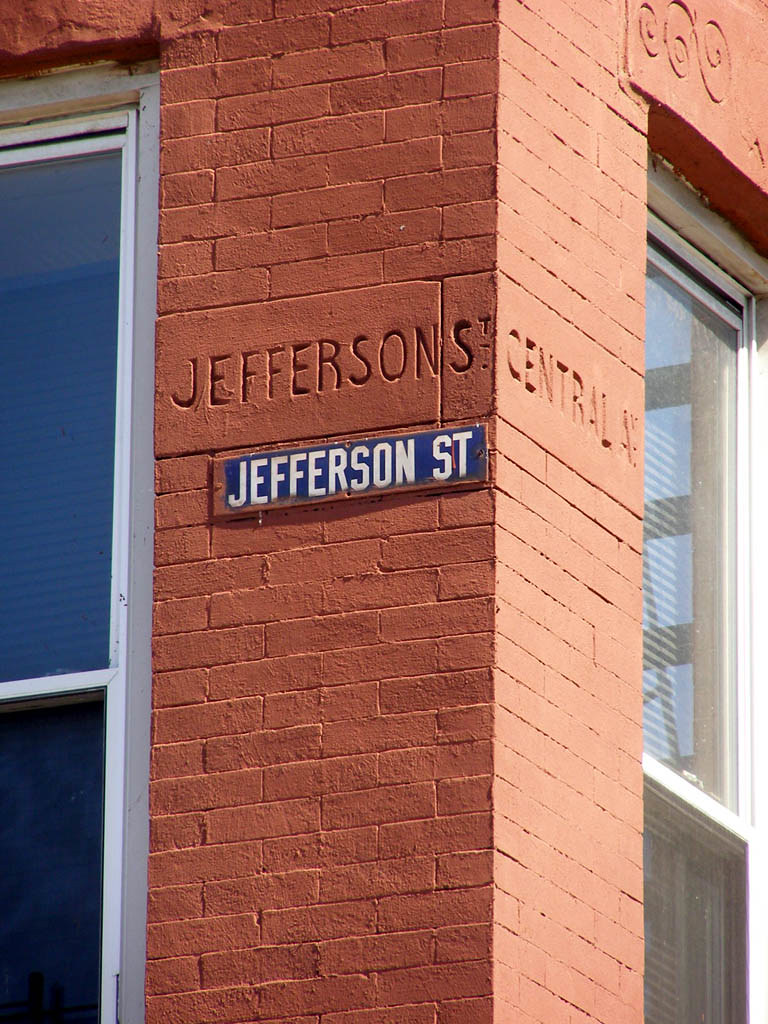The image features a red brick building situated at the intersection of Jefferson Street and Central Avenue. The building's corner is prominently displayed, with its red brick facade highlighted by the white trim around the windows. Each window is framed with metal, blending seamlessly into the building's classic architectural design. On the left side of the image, the camera captures the portion of the building facing Jefferson Street, while the adjacent side showcases Central Avenue. Above, a blue street sign with white lettering marks the intersection, mirroring the inscription of "Jefferson Street" directly etched into the brickwork of the building itself. Windows are visible on both sides of the structure before they extend out of the frame, adding to the building's overall charm and historical appeal.